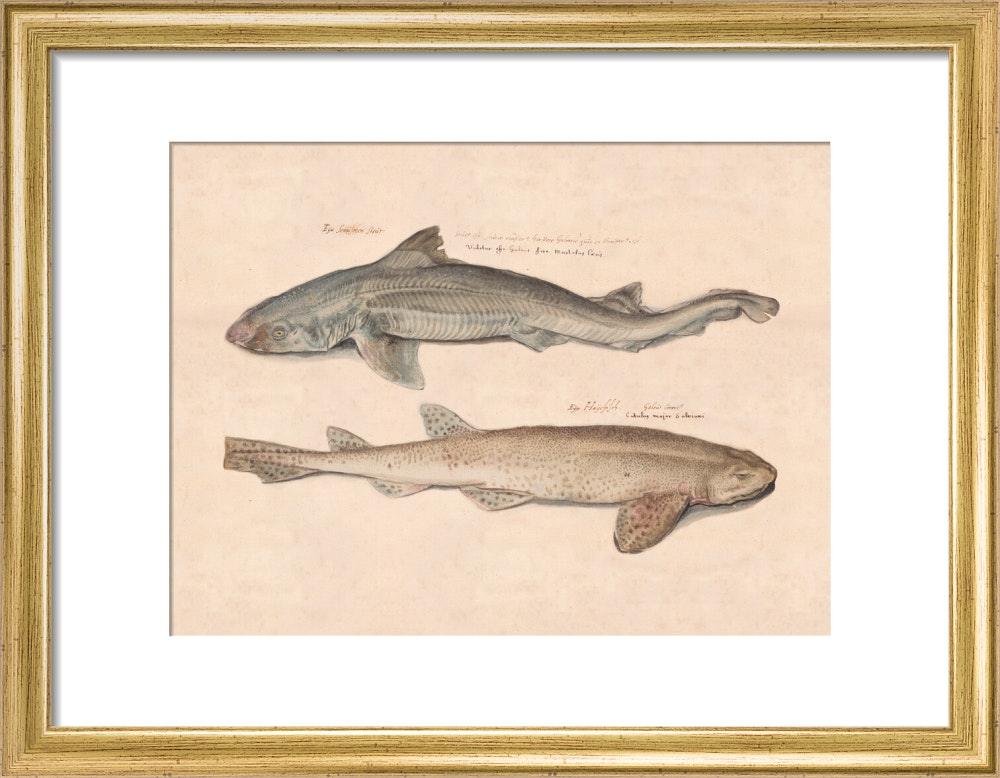The image captures a close-up of a framed piece of art, where the frame itself is made of light brown wood with a white inner border. The centerpiece is a detailed drawing on beige, aged paper that features two fish: a dusky smooth hound fish and a cat shark fish. The cat shark, located on the top, is rendered in various shades of gray, displaying intricate details including lines that run across its body. Below, the dusky smooth hound fish is depicted with a pattern of sand-colored spots along its back and fins, lightening to white on its underside. Both fish are oriented in opposite directions, with the cat shark facing left and the hound fish facing right. Handwritten text is situated above each fish, although it is somewhat blurry and unreadable. The image is well-lit with ample natural light, highlighting the clear and meticulous artwork within the frame.